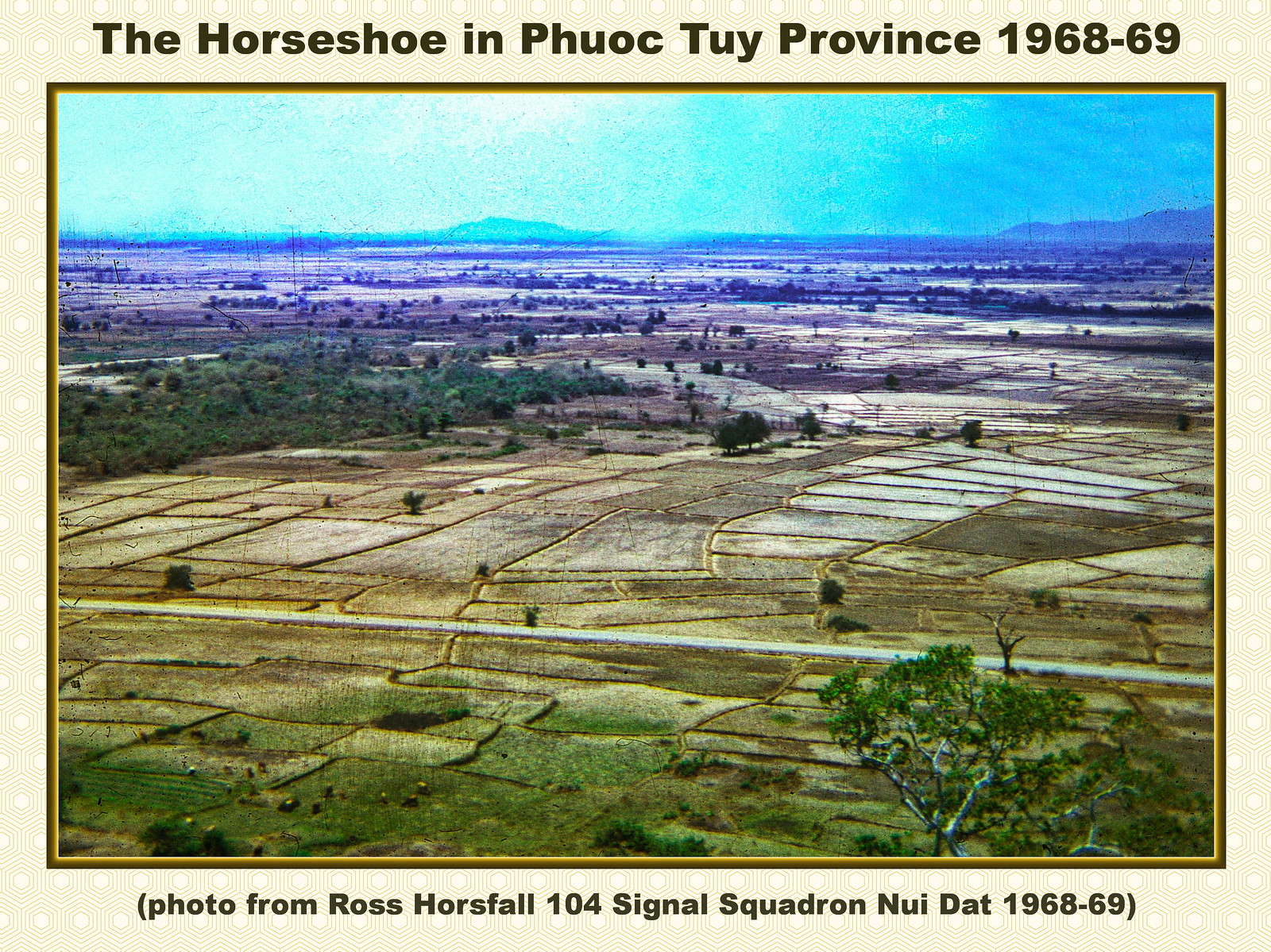The image showcases an aerial view of a rural landscape, prominently featuring farmlands divided into distinct plots, interspersed with sporadic trees and bordered by a mountainous horizon. The photograph, taken in Phuoc Toi Province, Vietnam, during the years 1968-69, is framed with a light yellow background adorned with small white polka dots. At the top of the image, bold sans-serif text states, "The Horseshoe in Phuoc Toi Province 1968-69," and at the bottom, smaller text reads, "Photo from Ross Horsefall, 104 Signal Squadron, Nui Dat, 1968-69." The photographic landscape, centered within a gradient tan or golden inner border, shows hues of tan, yellow, green, brown, blue, and light blue, reflecting an outdoor midday setting. Despite its age and some faded quality, the photograph clearly depicts the expansive, flat fields and distant mountains, under a partially clear sky.